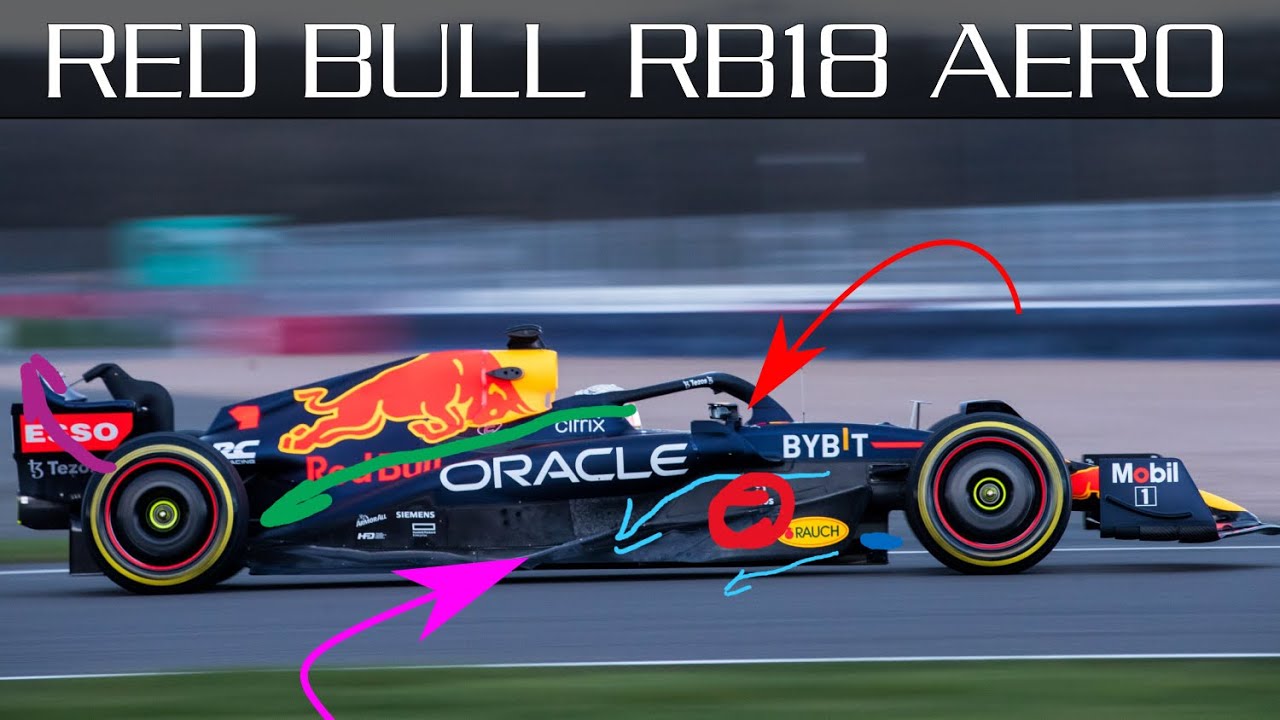The image is a highly saturated, vibrant photograph of a Red Bull race car, aggressively speeding to the right, evidenced by the blurred background. The top of the image features a black rectangle with white block text proclaiming "RED BULL RB18 ARROW" in all capitals. The car itself dons several logos, including a prominent Red Bull emblem, "Oracle" where the driver sits, "Bybit" just in front of the driver's seat, and "Mobil" on the front.

Additionally, the image has been edited to include various arrows and circles pointing to different parts of the car. A digitally created red arrow arcs around and highlights the driver's seat, while a pink arrow points to the car's underbelly. A green, digitally hand-drawn arrow indicates the back tire. There are also two thin blue hand-drawn arrows pointing to the undercarriage of the vehicle, and a purple, marker-like arrow aimed above the car's rear, not pointing to anything specific. A sloppily drawn red circle marks the midsection of the car, just in front of where the driver sits. The overall effect is a colorful and dynamic presentation that emphasizes different elements of the Red Bull race car.